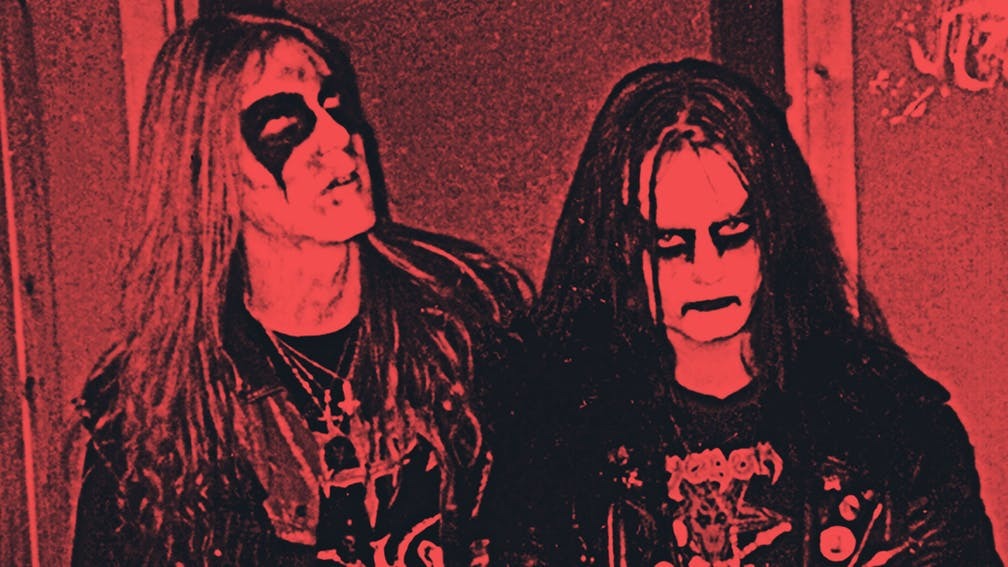This professionally taken, old photograph, now digitally enhanced, features an indoor scene of a defunct death metal band, marked by a striking red background that dominates the horizontally rectangular image with no border. The band members, shrouded in an eerie and dark aesthetic, stand out with their intense and dramatic appearance. The shorter musician, known by the moniker "Death," has long black hair and notably battled a mental illness that led him to believe he was dead – a tragic narrative explored in a documentary. The taller musician sports long blonde hair. Both are dressed in long black jackets and shirts, adorned with unique necklaces, and heavy black face paint around their eyes, enhancing their sinister, gothic look. Their expressions convey anger, further intensifying the overall haunting vibe of the photograph. A small, indistinct blob is visible in the top corner, adding to the image's mysterious ambiance.